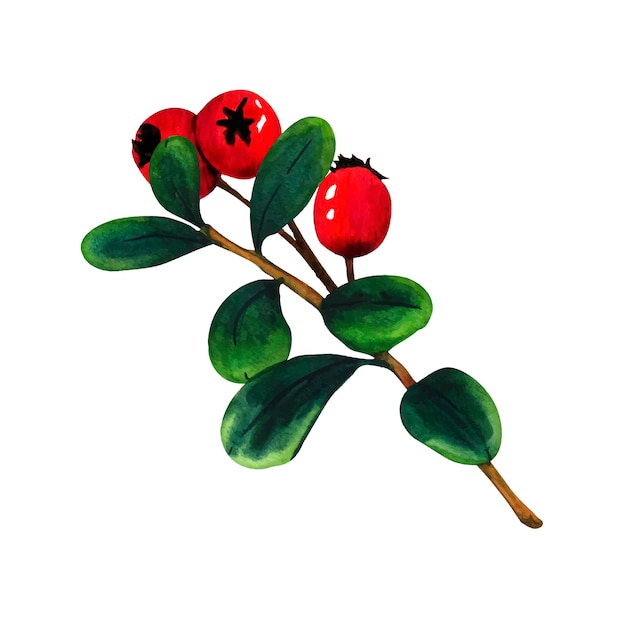The image is a detailed rendering, possibly a painting, of a plant against a stark white background. The plant features a singular brown stem that branches off into smaller twigs, each adorned with lush green leaves and striking red berries. The leaves, numbering around seven, are a muted jade green and have rounded, blunt tips reminiscent of a jade plant, although the plant itself isn't identified as one. The focal points, however, are the three large, shiny red berries. They are notably the size of plump grapes and have black ends, giving them a varnished appearance. These berries are attached to the twig-like branches by smaller, leafless stems. The vibrant juxtaposition of the green leaves and the glistening red berries against the plain white backdrop brings this image to life, emphasizing its artistic, almost surreal depiction.